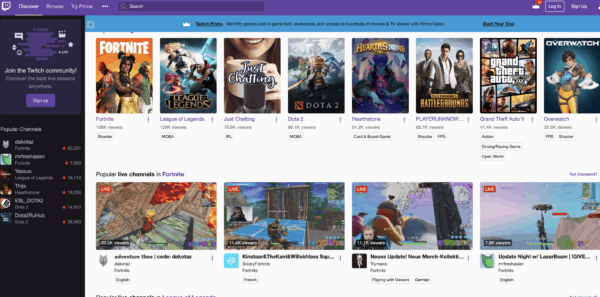**Screenshot of a Gaming Website Interface**

The image is a screenshot of a gaming website, showing a detailed layout with a white header at the top, containing white text and a search bar for easy navigation. Below the header, the main content area is divided into two sections. On the left, there is a vertical navigation column. The central area of the page features two rows of game thumbnails. 

At the top of the central section, a blue bar provides additional contextual information. The first row of game images includes popular titles such as "Fortnite" with an orange background, "League of Legends" (erroneously listed as "League of Nations"), "Just Chatting," "Dota 2," "Hearthstone," "Battlegrounds," "Grand Theft Auto V," and "Overwatch." 

The lower section of the page showcases a segment titled "Popular Live Channels in Fortnite," which contains four distinct images. These images depict various in-game scenes from Fortnite, including an intense battle scene and an underwater adventure, providing viewers with a vivid glimpse into the diverse gameplay experiences available in Fortnite.